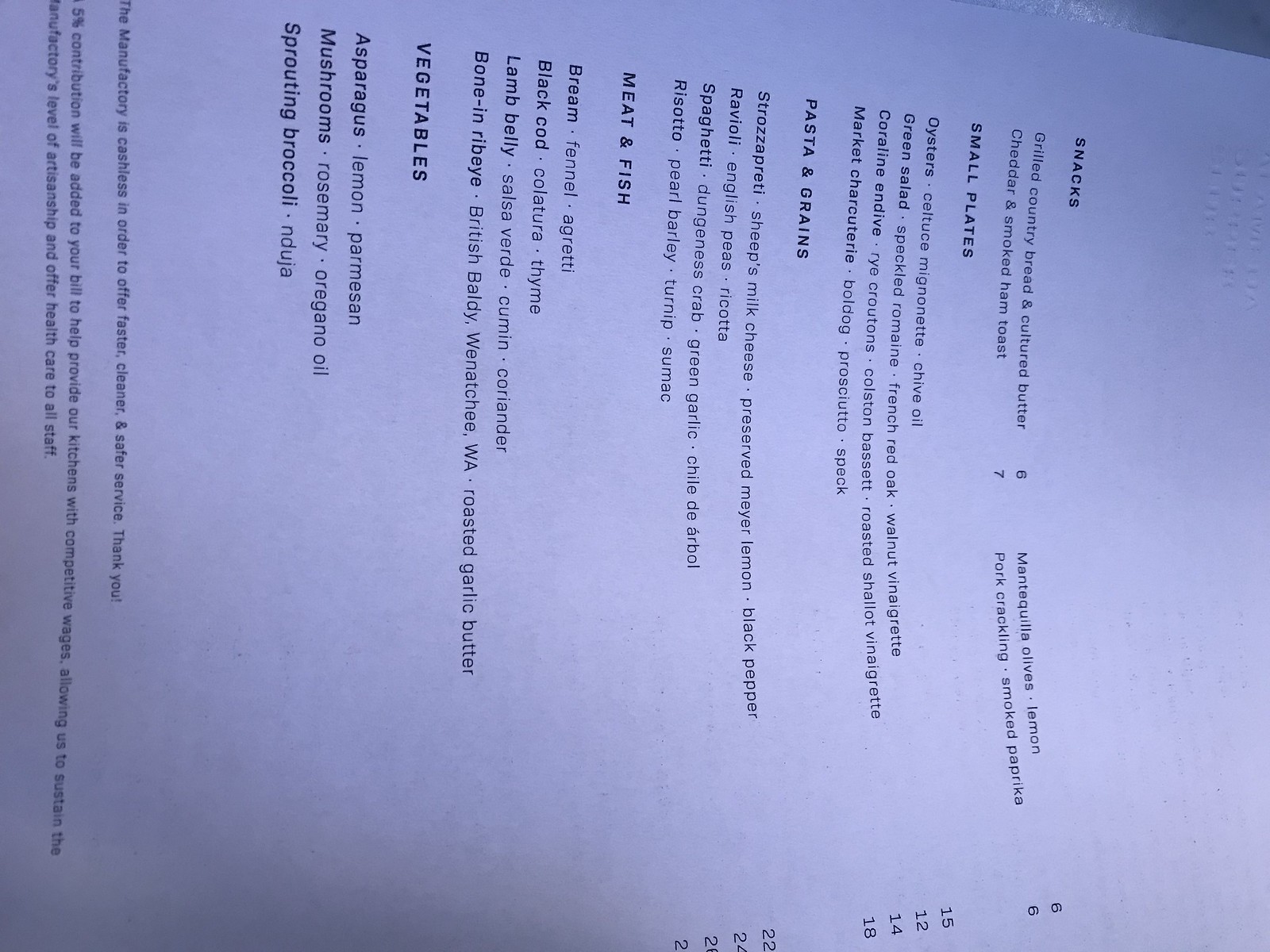The image captures a slightly tilted, poorly lit menu printed on white paper with black lettering, exhibiting a bluish hue due to the lighting. The menu is divided into several sections, each listing four options, starting with "Snacks" at the top, followed by "Small Plates," "Pasta and Grains," and "Meat and Fish." The "Veggies" section lists three options. There is no logo visible on the menu. At the bottom, partially cut off, is a notice indicating that the establishment is cashless for improved cleanliness and speed, along with other disclaimers.